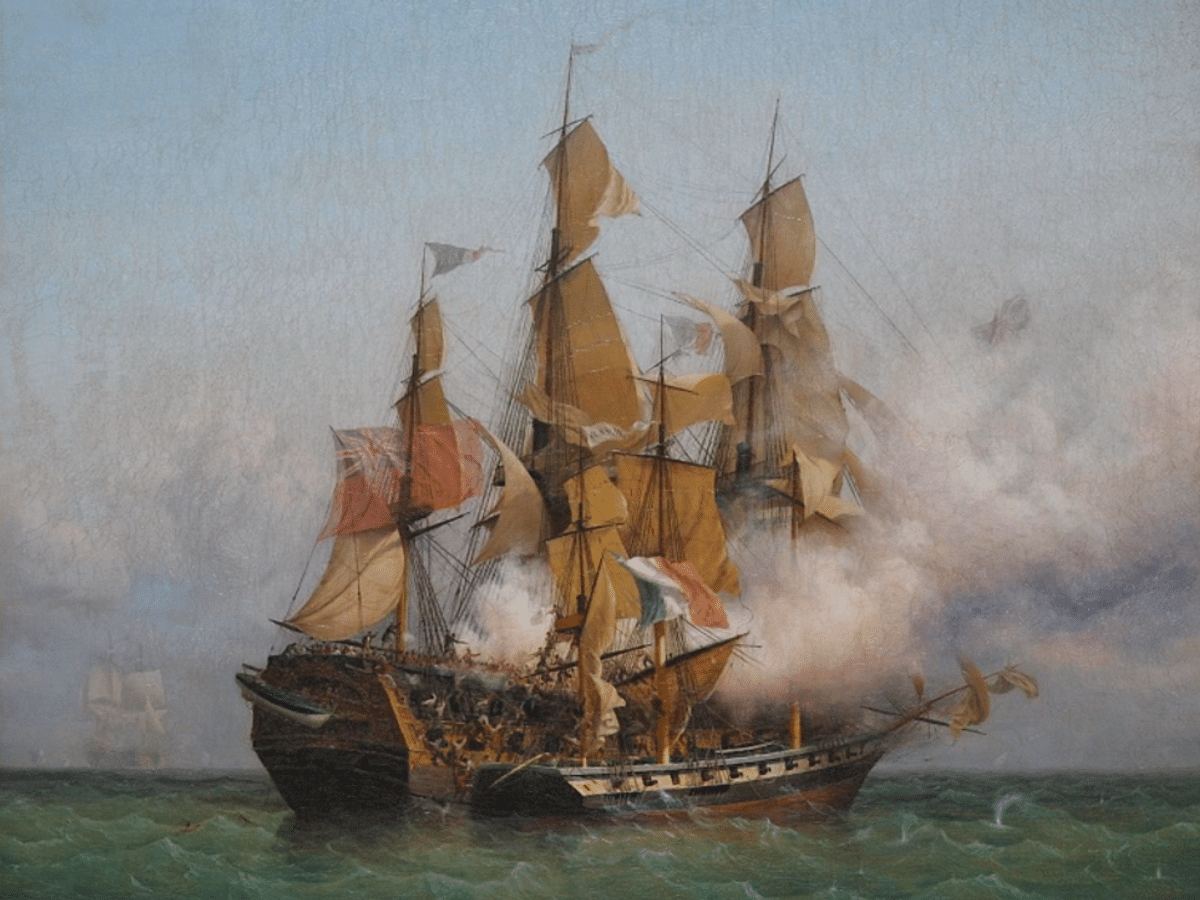This is an acrylic painting of a large, vintage wooden ship, prominently displayed in the foreground. The ship is adorned with multiple white sails billowing in the wind and features a red and blue flag at its front. The vessel's complex structure includes angular, round, and rectangular forms, making it an imposing sight. Tiny figures can be seen crawling along the sides of the ship, emphasizing its immense size. The sea beneath the ship is a murky green with light waves, suggesting a calm yet choppy surface. Clouds and possibly smoke fill most of the powder blue sky, adding a dramatic effect. In the background, on the far left, a faint outline of another ship can be discerned, blending into the horizon. The overall scene evokes a historical atmosphere reminiscent of colonial or pirate voyages.